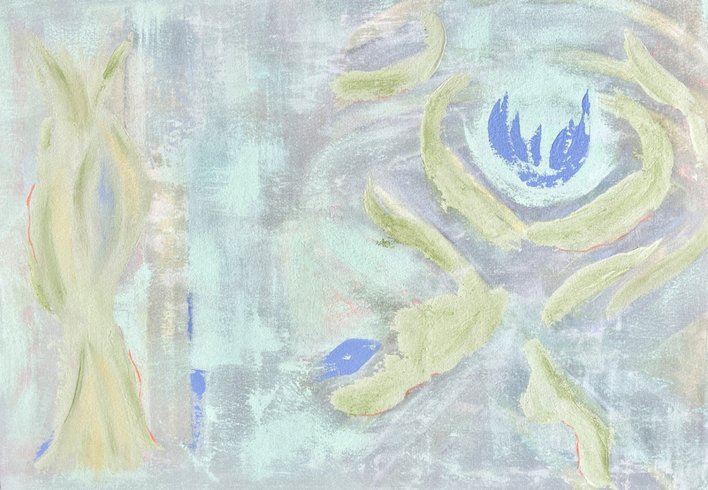In this abstract, pastel landscape painting, the background features a soft blend of light greens and grays, reminiscent of a sanded, sparse texture. Upon closer examination, the left side reveals a greenish stem that swirls upwards in a criss-cross pattern, evocative of organic growth. To the right, a captivating focal point emerges—a blue flame-like figure, which is set against a rich blue backdrop and surrounded by light green and white hues that encircle it.

Overall, the painting is composed of broad brush strokes that create the illusion of lily pads floating in a serene pond, reminiscent of Monet’s dreamy textures but with a modern, abstract twist. Scattered throughout, green and light green shapes resemble fish-like forms swimming amongst the abstract, almost graying cactus-like imagery. The composition combines touches of sky blue, off-white purple, and gray to enhance the ethereal quality of the scene. Poised above and slightly encircling these shapes is a flower-like figure, painted in shades of blue, its petals seemingly unfurling and emitting a gentle light bluish glow.